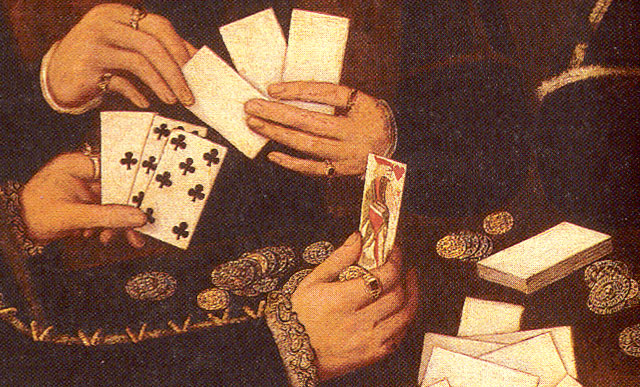The painting is an old, highly detailed depiction of people playing cards, focusing solely on their hands and the table. The image is horizontally rectangular with a predominantly dark brown palette, giving it a vintage and grainy appearance. The background is a dark brown, blending seamlessly with the players' dark brown clothing that reflects an old 17th-century style, characterized by intricate sleeve patterns.

The composition features four white, Caucasian hands prominently displayed. On the left side of the painting, a close-hand sports a ring and holds either a Jack or King of Hearts in one hand, with the other hand clutching three club cards devoid of numbers. Another smaller hand in the upper left corner also has two rings and holds three white-backed cards whose faces remain unseen. In contrast, the lower right-hand corner showcases a collection of these white cards scattered around, alongside numerous round coins or poker chips in dark colors with white flecks.

Overall, the painting immerses the viewer in a scene of an intense, historical card game, capturing minute details of the players' hands, the cards, and the cluttered tabletop, thus highlighting the tension and strategy of the moment.